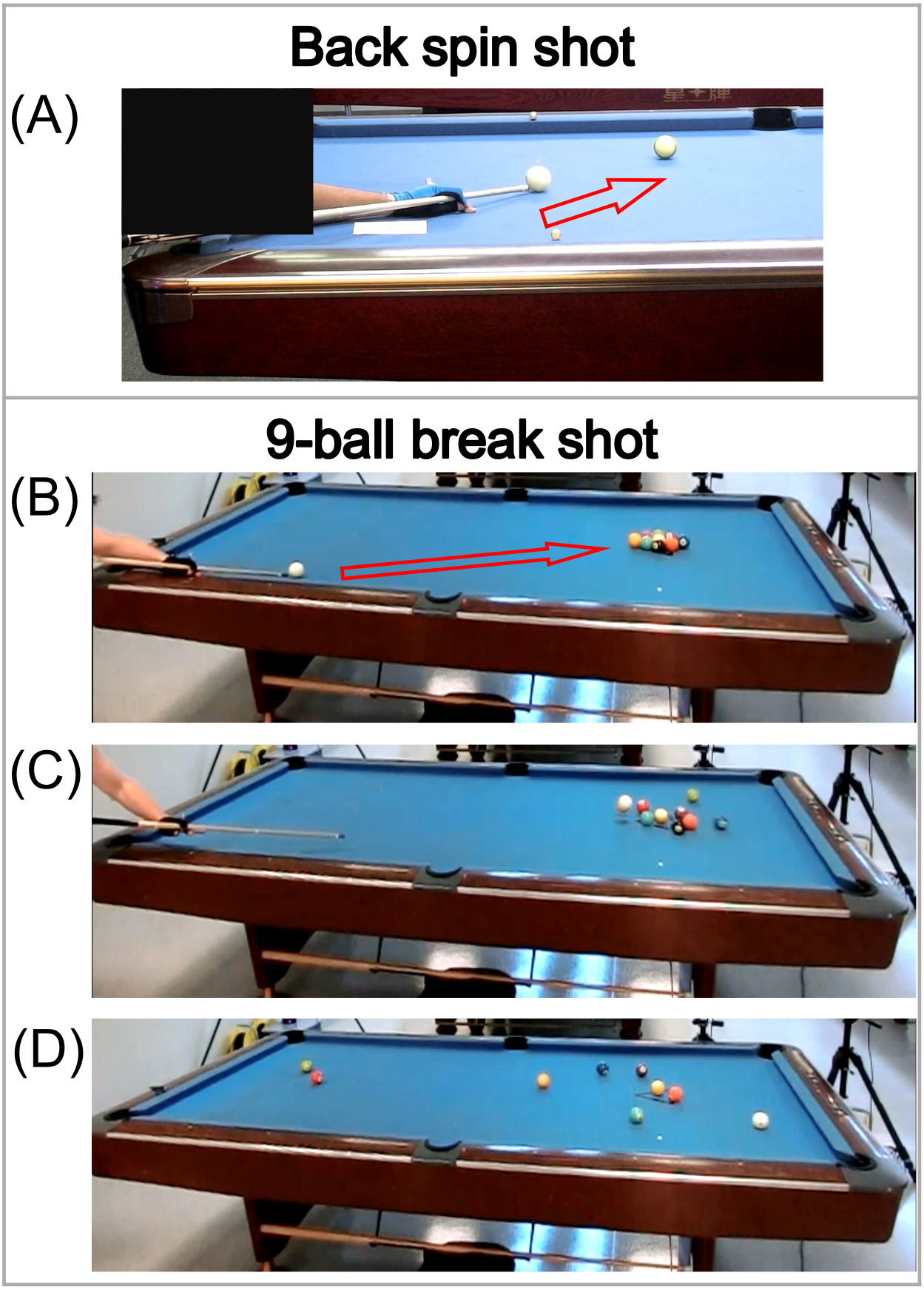The image is an instructional breakdown for playing pool, divided into four labeled sections: A, B, C, and D. Each section is a color photograph of a pool table with a blue felt surface and a brown wooden outline, with the cream-colored holes visible in various locations. 

**Section A**, labeled "Back Spin Shot," shows a close-up of a pool cue aimed at the white cue ball, held by a hand wearing a light blue glove. An overlaid red arrow indicates the intended direction of the shot aimed toward another pool ball with red accents. The player’s face and body are censored with black squares, drawing focus to the positioning and technique of the shot.

**Sections B, C, and D** are collectively titled "Nine-Ball Break Shot." 

- **Section B** shows the initial break setup, with the player's gloved hand aiming the cue at the clustered multicolored balls in the center of the table. Another red arrow overlays the image to illustrate the direction of the cue ball's impact.

- **Section C** captures the moment just after the break, with pool balls slightly blurred, indicating their motion as they scatter across the table.

- **Section D** depicts the final positions of the scattered balls post-break. Specific colored balls—such as an olive, orange, yellow, dark blue, light blue, purple, and more—are dispersed around the table, demonstrating the result of a successful break shot.